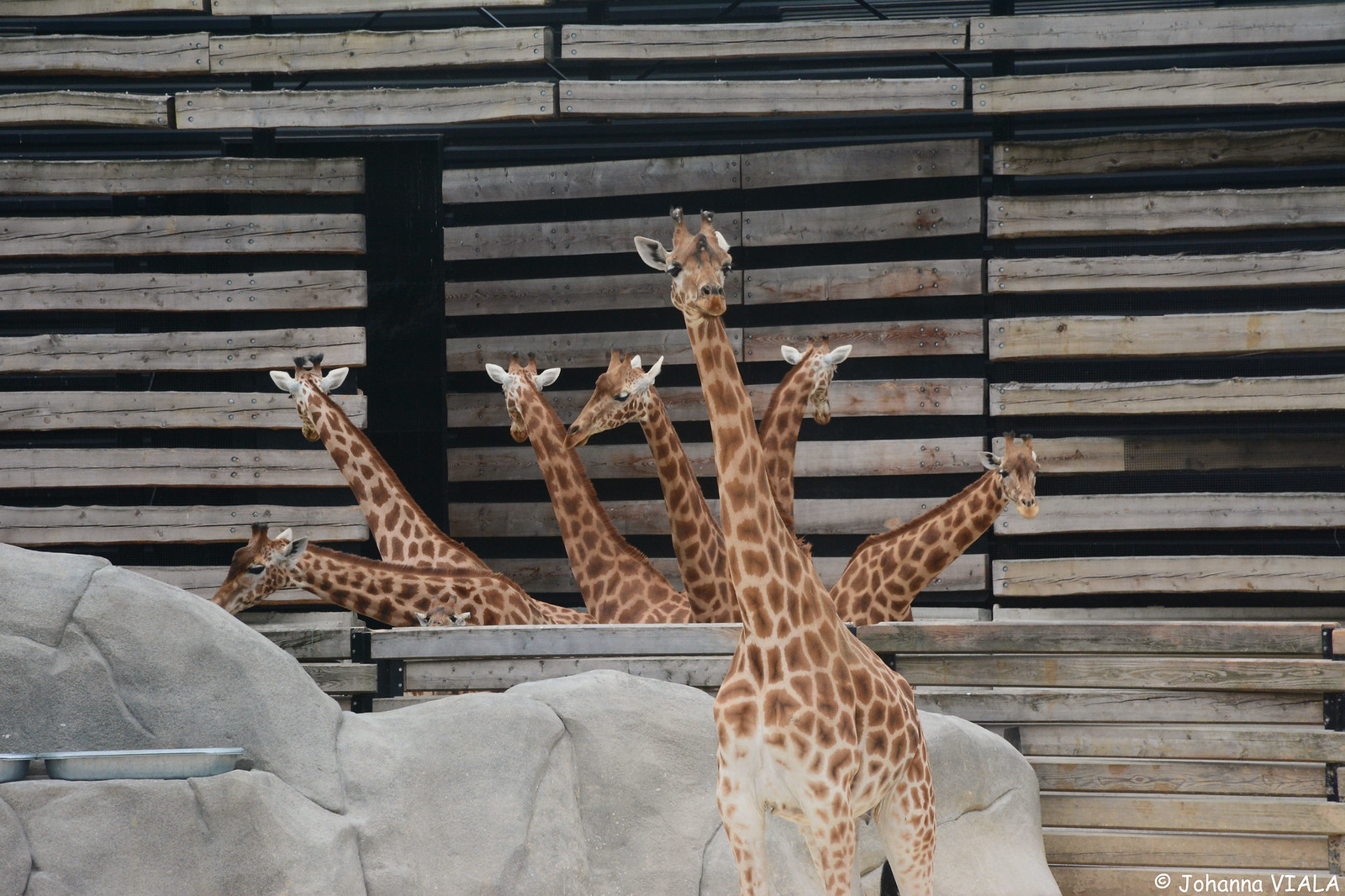The photograph captures a zoo enclosure featuring a group of seven giraffes. Dominating the centre, a giraffe stands in the foreground, prominently displaying its brown and off-white patterned body. This giraffe, only visible down to its knees, engages the viewer with its gaze directed towards the camera. Surrounding it are artificial gray boulders, adding to the zoo-like ambience. On these rocks, there are two metal pans, possibly for feeding or watering the animals.

Behind the foreground giraffe, a series of wooden barriers horizontally span the enclosure, interspersed with slightly varied colored planks – some lighter and others darker brown, even streaked with black. The giraffes positioned further in the background are divided by these barriers, only their long necks and heads visible as they peek over. These six giraffes reveal varied patterns, some with lighter hues compared to the giraffe in the foreground. 

The environment is further framed by additional horizontal wooden beams that form the backdrop, contributing to the enclosure's aesthetic. In the bottom right corner of the image, a white copyright mark reads "© Johanna VIALA," indicating the photographer's ownership. This meticulous composition not only showcases the majestic giraffes but also highlights the detailed design of their zoo habitat.